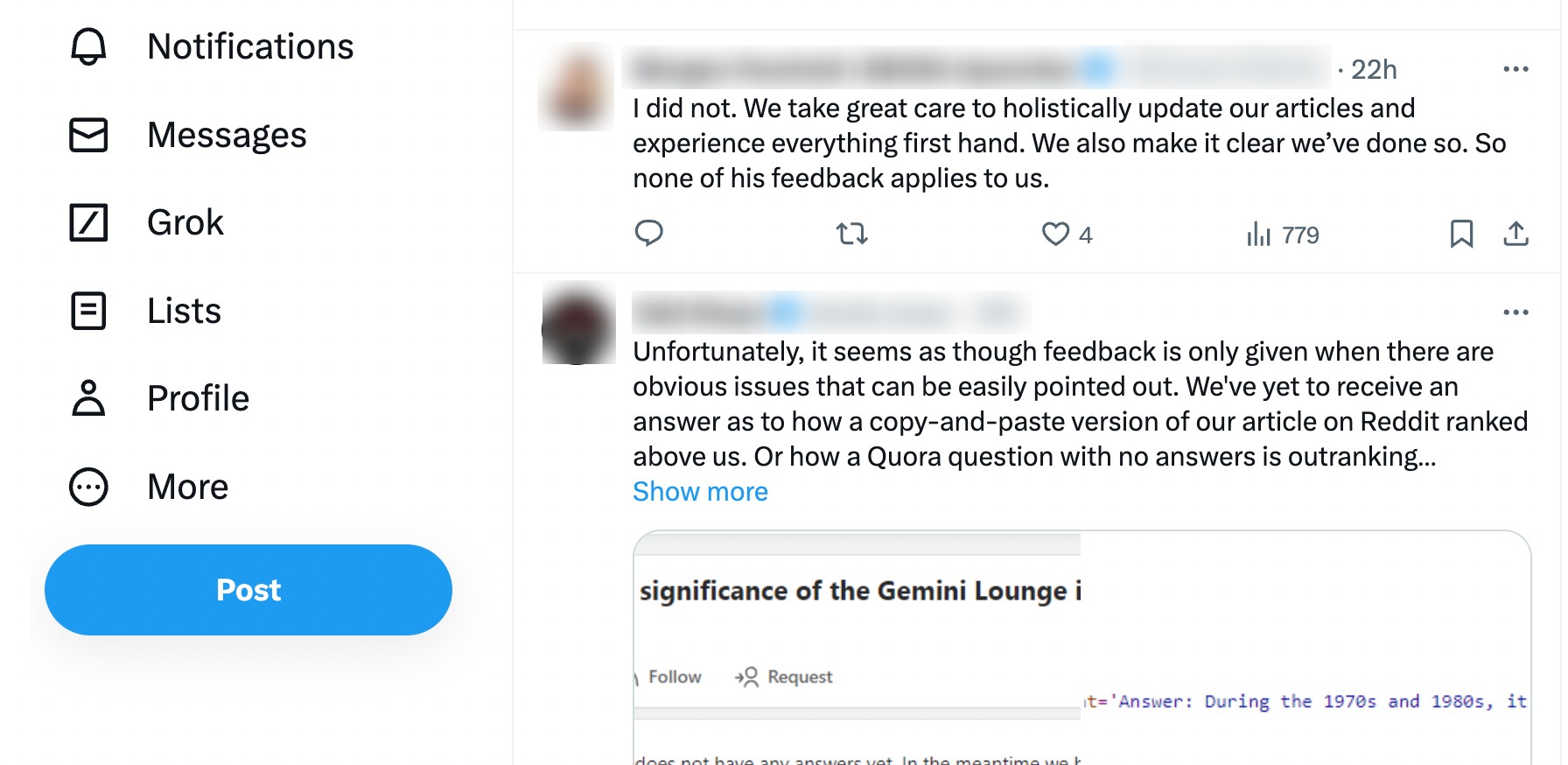The image displays a user interface layout. On the left side of the screen, there is a menu with several options: "Notification," "Messages," "GROK," "Lists," "Profile," and "More." Below the menu, there is a prominent blue button labeled "Post." 

On the right side of the screen, there are two blurred-out profile pictures and names. The first blurred profile shows a time stamp of "22 hours" and a comment that reads: "I did not. We take great care to holistically update our articles and experience everything first-hand. We also make it clear we've done so, so none of his feedback applies to us." This comment has received four likes, bringing the total to 779 likes.

Below this, there is another blurred-out profile with a comment stating: "Unfortunately, it seems that the feedback is only given when there are obvious issues that can be easily pointed out. We've yet to receive an answer as to how a copy-and-paste version of our article on Reddit ranked above us, or how a Quora question with no answer is outranking..." This comment cuts off with an ellipsis, and a blue hyperlink below it reads "Show More."